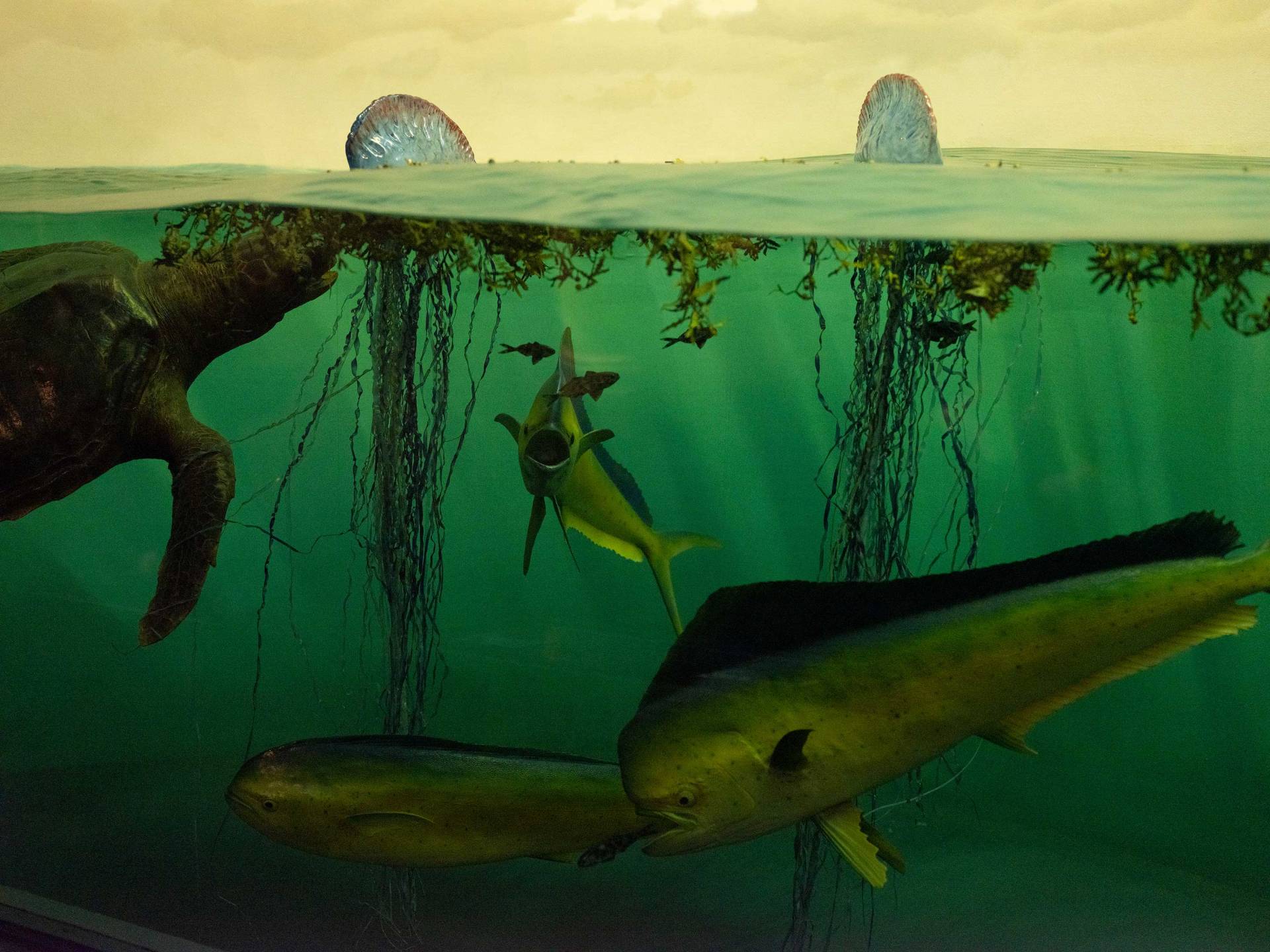This detailed illustration, likely computer-generated due to its photorealistic quality, depicts a rich underwater scene that highlights both the underwater and above-water environments. The water is a vibrant green, giving a distinct impression of seawater. Above the surface, the weather appears overcast with a gray sky, and two large blue seashells can be observed at the water's edge.

Underneath the water, a detailed array of sea life is visible. Dominating the scene is a large turtle, or possibly a tortoise, positioned on the left, who appears to be swimming and nibbling on some green, moss-like sea vegetation hanging down from the surface. Surrounding the turtle is a vibrant community of smaller black fish, some of which seem endangered by an open-mouthed shark with a pointy nose, appearing poised to attack.

Adding to the depth of the environment, there are three very large, elongated fish with bumpy heads, exhibiting a greenish-beige tone with golden-yellow highlights and a distinctive long dorsal fin stretching from head to tail. These fish are seen motionless in the background, blending harmoniously with the overall green-tinted underwater scene.

The underwater flora is detailed, with black roots and stringy sea plants contributing to the lush ecosystem. This vivid and intricate scene masterfully captures the dynamic interplay between marine life and their habitat.